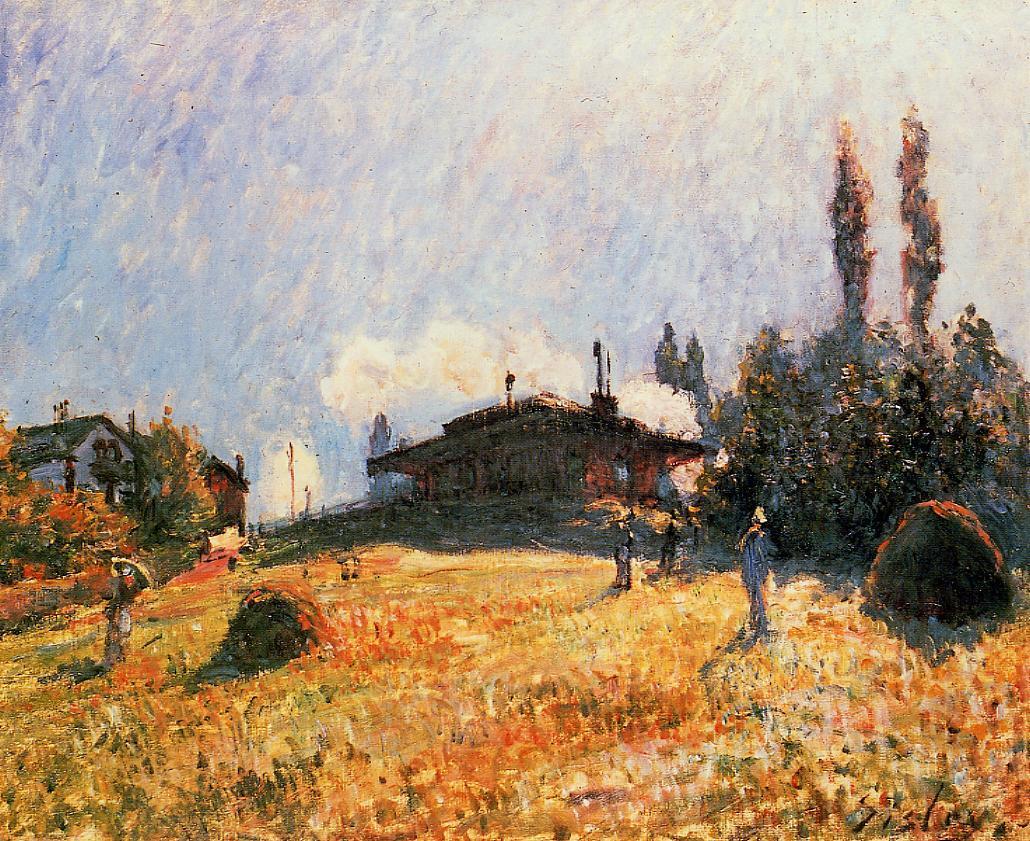This vibrant impressionistic painting captures a rustic rural scene with a field, likely a hay field, rendered in a mix of bright orange, pale blue, pastel blue, pink, white, and green hues. The field, appearing somewhat blurry, features the indistinct shapes of four people amidst tall blades of hay. Central in the composition is a brown house, flanked by another smaller white house with a green roof to the left. The landscape also includes two prominent trees and various bushes and shrubbery, particularly behind a haystack on the right. Above, the expansive sky teems with blue, pink, and white dots representing clouds, complemented by large, billowy white clouds. The entire scene is depicted in a choppy, impressionistic style that gives the painting its blurry, almost crayon-like texture, making definitive details hard to distinguish.